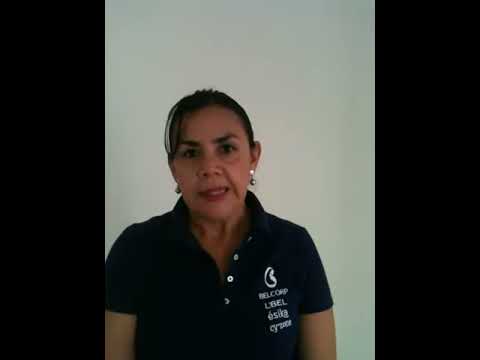The image appears to be a slightly out-of-focus and horizontally rectangular screenshot from a video. It features a woman, likely in her 40s, standing in front of a light blue or off-white background. The image includes thick black borders on the left and right sides but none on the top or bottom. The woman has dark hair, swept back with a few strands falling across her forehead, and she is wearing gold earrings. Her outfit is a dark blue, short-sleeved, polo-style button-up shirt, displaying a white logo over her left breast that seems to say "Bell Corp" with additional unreadable white text underneath. The woman, who seems to be Hispanic, is partially open-mouthed as if speaking, suggesting she might be mid-sentence in a video, possibly for a work training or YouTube announcement.